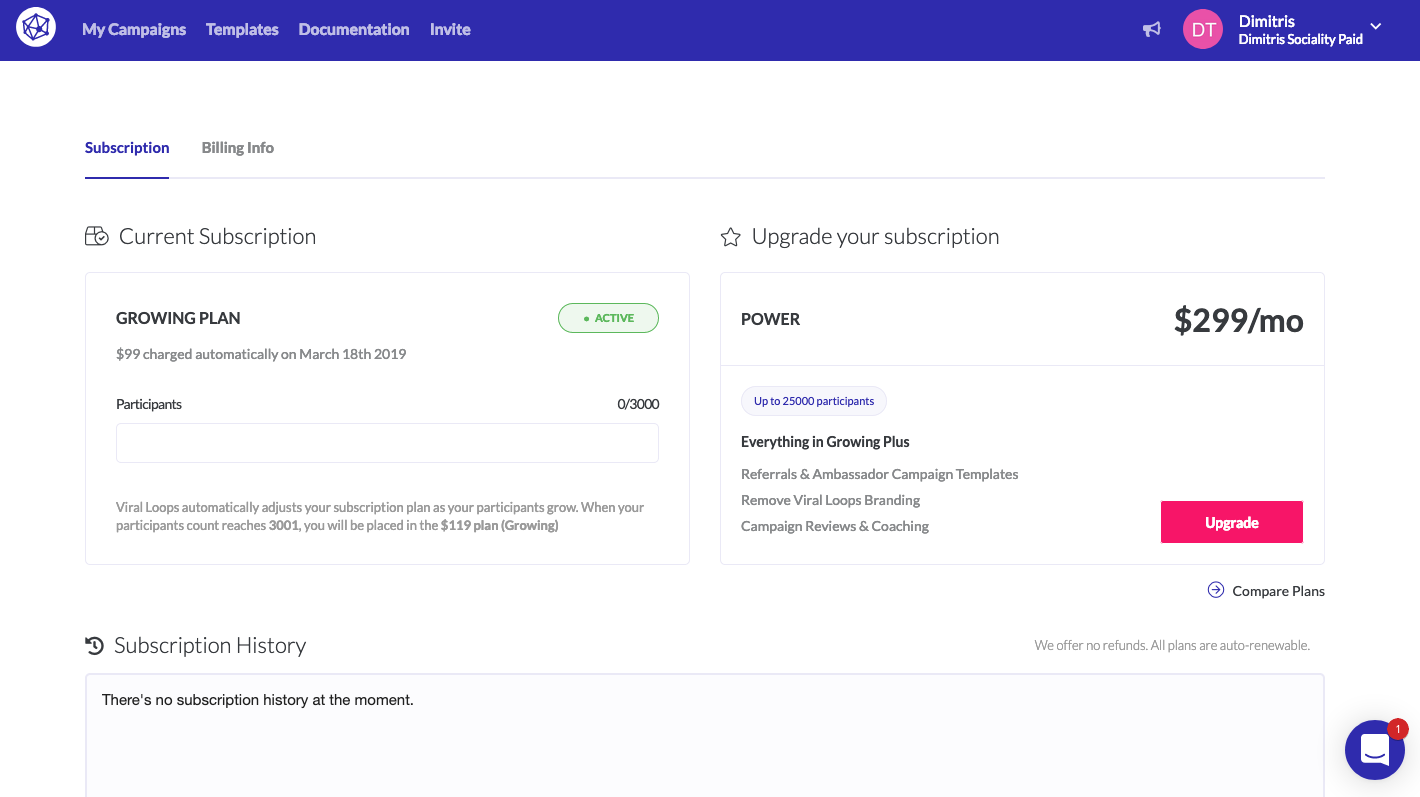The image shows a detailed view of Dimitri’s social platform subscription page. The header of the page is blue, and there are several tabs located at the top left corner: 'My Campaigns,' 'Templates,' 'Documentation,' and 'Invites.' On the top right, a user profile icon labeled "DT" indicates that the page belongs to Dimitri.

The lower section of the page transitions to a white background. Two primary tabs are visible: 'Subscription' and 'Billing Info,' with 'Subscription' being highlighted in blue and 'Billing Info' appearing in raised grey. Detailed subscription information occupies the main section of the page. 

A segment titled "Current Subscription" indicates Dimitri is on the "Growing Plan" with a $99 charge automatically applied on March 18, 2019. The status is marked as "Active," demonstrated by a green button labeled "Active." There's a section for participants, which is currently empty. Beneath this, a note explains that Viral Loops charges are added to the subscription plan as participant numbers grow. It advises that upon reaching 3,001 participants, the user will transition to the 2019 Growing Plan.

At the very bottom of this section, "Subscription History" is indicated, showing no subscription history at the moment. On the left side of the page, there’s an option to upgrade the subscription to the "Power" plan for $299 per month, covering up to 25,000 participants. This offer is written in blue text adjacent to a description in a black tag detailing the benefits of upgrading: "Everything in Growing plus, Reference and Ambassador Campaign Template, Remove Viral Loops Branding, Campaign Reviews, and Coaching." A pink 'Upgrade' button is located below this description.

Additionally, a note at the bottom of the page states, "Compare Plans. We offer no refunds. All plans are auto-renewable." A blue and white chat button with a red notification mark is situated in the bottom right corner, indicating one unread message.